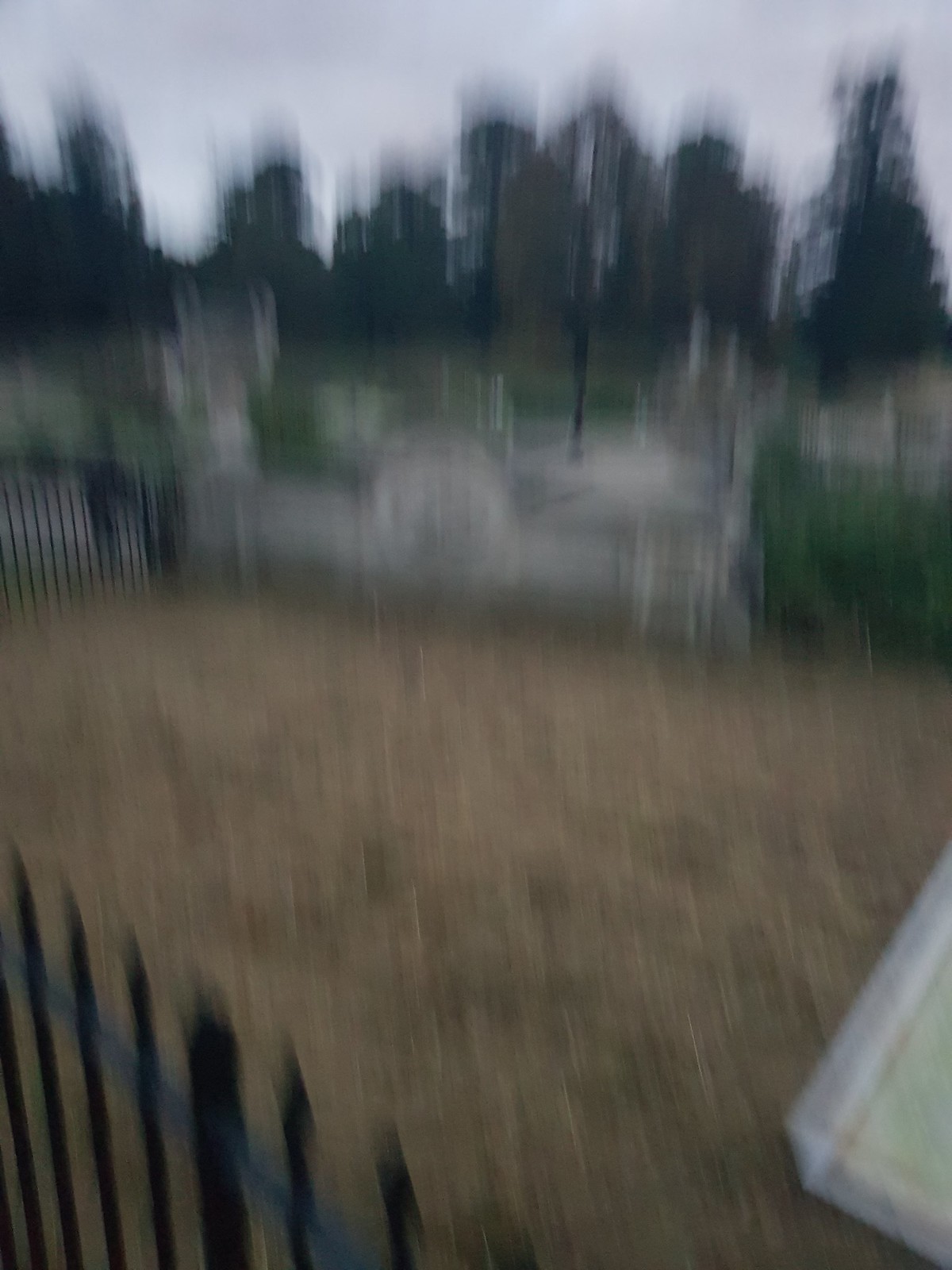The image, captured from a first-person perspective and likely in motion, is very blurry. It depicts an outdoor scene featuring a black, pointed iron fence that appears on both the left and right edges of the photograph, suggesting the viewer is positioned behind this fence. The ground immediately beyond the fence consists of either brown, dead grass or dirt. Scattered green bushes are visible amidst this background.

Further into the image, a whitish-gray sky looms over the scene, indicative of a cloudy day. There are multiple trees, both in the foreground and as a distant tree line, though their details are indistinct due to the blur. To the right, at the bottom corner, there is a square white object, which could be part of a bench, a directory, or another structure.

Central to the image is a pathway, perhaps a sidewalk or a concrete divider, weaving through the scene. This pathway is flanked by patches of grass and occasional trees. Despite the motion blur, the outdoor setting suggests it could be part of a park, cemetery, or enclosed section of a residential area.